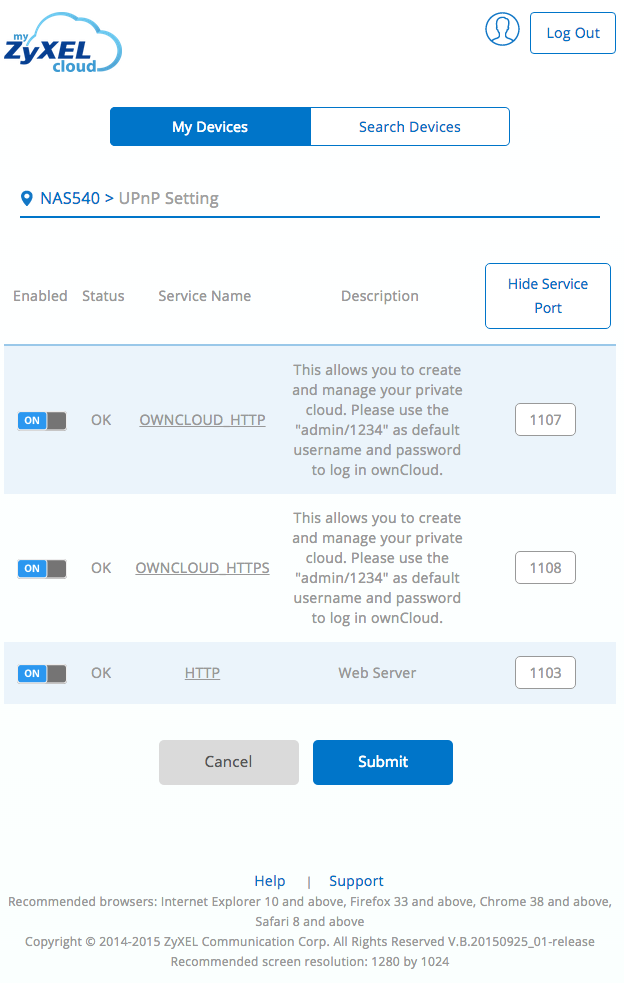**Detailed Caption**:

This image is a comprehensive screenshot of the settings page on the My Zyxel Cloud website. At the top left corner, there's a cloud logo outlined in blue with the text "My Zyxel Cloud" inscribed within it. The word "Zyxel" is uniquely stylized, featuring a capital 'Z', lowercase 'y', and then capital 'X-E-L'. This logo is positioned in the lower left portion of the cloud icon.

In the top right corner of the page, a blue profile picture icon is displayed. To its right, there's a white button with a thin blue outline featuring blue text in the center that reads "Log Out".

Central to the page are two connected buttons. The left button is blue with white text that says "My Devices" and has slightly rounded corners. Adjacent to this, the right button is white, also with a thin blue outline and blue text reading "Search Devices", featuring rounded corners as well.

Below this section, on the left side, there is a blue geolocation pin icon. Next to it, in all caps blue text, is the label "NAS 550". To the right of this label, a blue arrow points to text in light blue or light gray reading "UPnP Setting". This section is separated from the main body of the page by a medium-width blue line.

The main body is organized into rows. The first row is quite wide and serves as a header, featuring light gray text that labels the columns: "Enabled", "Status", "Service Name", and "Description". To the right, there is a white button outlined in blue with the text "Hide Service Port" in the middle.

Following this, each row alternates between a light blue and white background. The first row with a light blue background has a toggle button set to "On", displayed as a blue rectangle with white text "On" next to a gray rectangle. The "Status" column contains light gray text reading "OK". Under the "Service Name" column, the text "Own Cloud HTTP" is underlined in gray. Descriptive details are listed to the right. 

At the bottom of the page, there are two buttons: a gray button on the left with dark gray text that says "Cancel", and a blue button on the right with white text that says "Submit".

This image offers a detailed view of the configuration options and interface layout for managing devices and services within the My Zyxel Cloud platform.